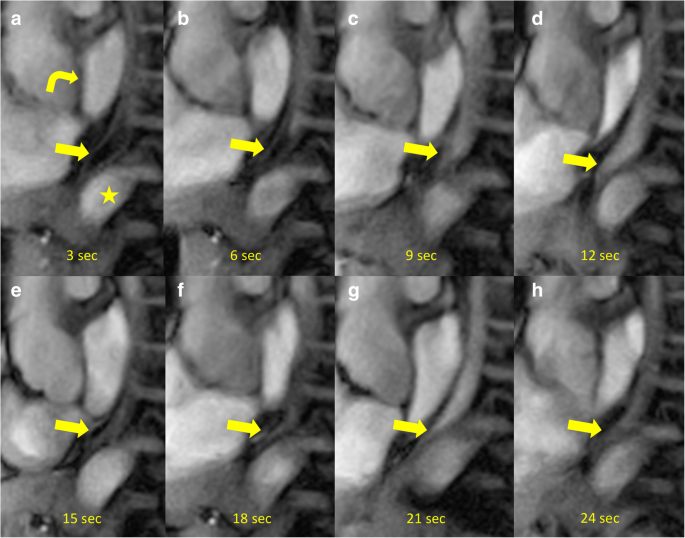This is a sequence of eight black-and-white medical imaging photos, labeled from 'a' to 'h,' showing either x-rays or CT scans. These images are arranged in two rows, with 'a' to 'd' on the top row and 'e' to 'h' on the bottom. Each image is marked with a series of timestamps: 3 seconds, 6 seconds, 9 seconds, 12 seconds, 15 seconds, 18 seconds, 21 seconds, and 24 seconds. The images feature yellow arrows pointing to specific areas, guiding the viewer's attention to details that change or progress over time. Additionally, a yellow star marks a focal point in each image, which could indicate a significant finding such as a tumor or a moving object within the body, possibly being tracked through the digestive tract. The precise nature of the subject in the images is unclear, but it appears to involve internal tissue, possibly bone or organs, demonstrating some notable change or movement as time progresses.